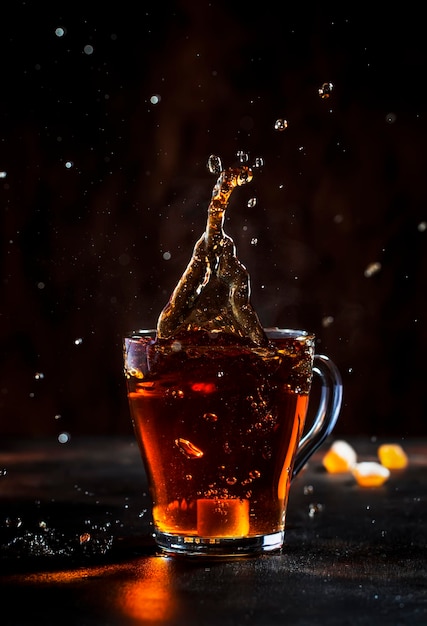This vivid photograph captures the dynamic moment when a clear glass mug, filled with a rich amber or deep golden-brown liquid that resembles beer or hard liquor, is forcefully slammed onto a black surface. The impact launches the liquid high into the air, creating a striking splash that arcs outward in a triangular shape. Droplets and beads of liquid are suspended mid-air, their motion illuminated by a light source off to the right of the image, adding a sparkling effect to the scene. The background is dark and blurred, suggesting a nighttime setting, which enhances the clarity and drama of the splash. Scattered in the background to the right are a few ice cubes, seemingly made out of the same golden liquid, and there are indistinct shapes that could be food items like nuts or candy. The overall composition is energetic and visually captivating, making it look like an advertisement for a spirited beverage.